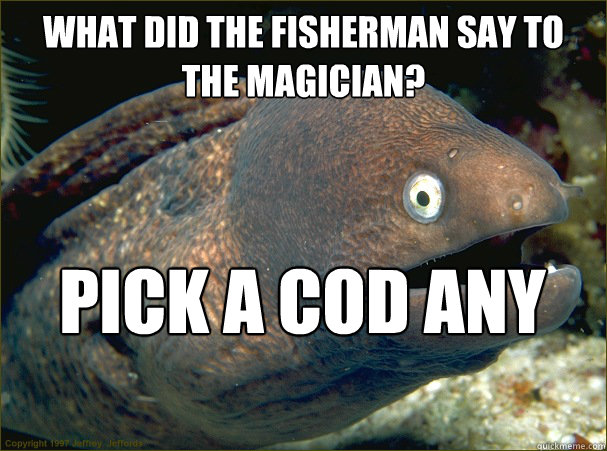In a detailed scene, a very muscular man, almost fully naked save for black underwear with thigh straps, poses on a bed in a kneeling, crouched position. He's staring intently at the camera, showcasing his bald head contrasted by a grayish beard and mustache. Notably, he bears a large, dark tattoo on his upper right arm. In front of him lies a cylindrical black bag adorned with a white ribbon, which he appears to be straddling. The bedding beneath him features a camouflage pattern of red, gray, black, and white colors, while the headboard is dark brown with matching posts. The surrounding wall is textured black. The pillows, made of black leather with white ribbon accents, complement the bed setting. Additionally, a white outlet or light switch is visible near the bedposts. Centered at the bottom of the image, large white block letters spell out "HAI."